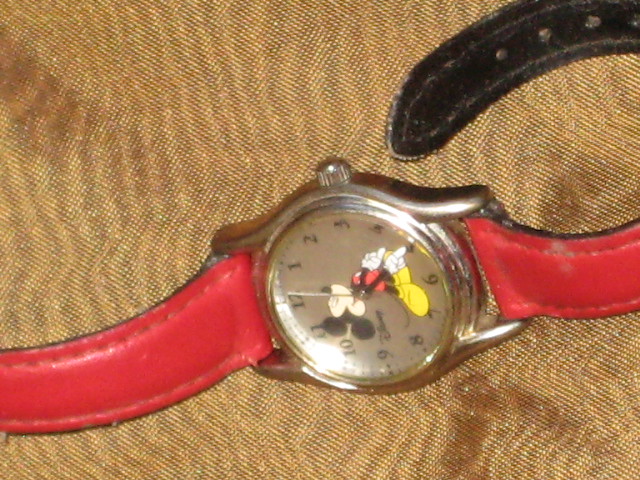This is a detailed close-up photograph of a worn, vintage-style child's wristwatch featuring a picture of Mickey Mouse on its clock face with the Disney logo next to him. The watch has a red leather strap, worn and faded with red on the top and brown below, and the watch itself has a stainless steel frame and a silver-toned dial on the right side. The clock face shows a time of 10:00 with the short hour hand and long minute hand pointing at 10 and 12, respectively, although another interpretation shows Mickey's arms pointing to 4 and 5 with the second hand at 12, likely due to lens distortion or a different angle. Mickey Mouse, donning his classic red romper, yellow shoes, and white gloves, is looking to the right. The watch is lying on its side against a slightly wrinkled, rough-textured orangey-tan fabric with lighter brown lines running through it, which provides a unique rustic backdrop to the timepiece.